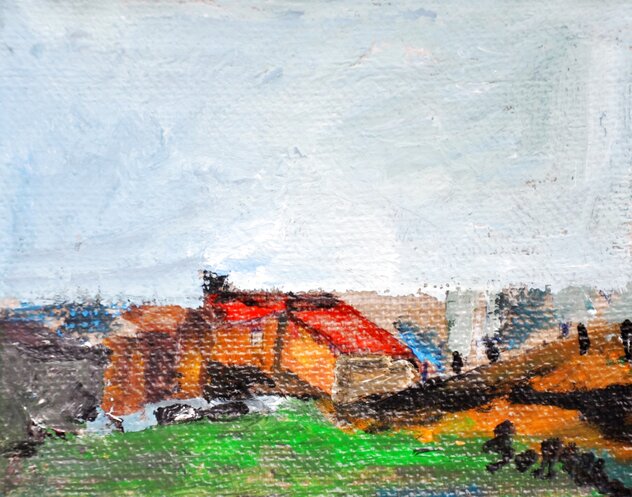The image is a photograph of an outdoor impressionist painting on a rectangular canvas, depicting a small town. The painting's top half is dominated by a sky that transitions from light blue to gray with subtle white brush strokes. Just above the horizon, which is brown, the sky displays varying shades of blue and gray. 

At the center of the painting, there is a focal point of three small, single-story, orange houses with red roofs. The house on the left simply appears orange, while the central house features a distinctive sloped red roof and a single white window with a black border. This house connects to another structure forming an L-shape, emphasizing the architectural details. 

In the foreground, there is a lush, green field that stretches toward the houses. The bottom right-hand corner of the painting contains several black blobs, likely representing trees, but no discernible text. Additionally, this corner might also display the artist's signature, although it is ambiguous and could just be more abstract forms.

On the left side of the painting, gray paint creates abstract shapes, while a small green hill with dark colors adorns the bottom section of the painting, creating a contrast with the bright green grass and enhancing the depth of the scene. The entire painting encapsulates a tranquil, rural atmosphere with its blend of natural and structural elements.